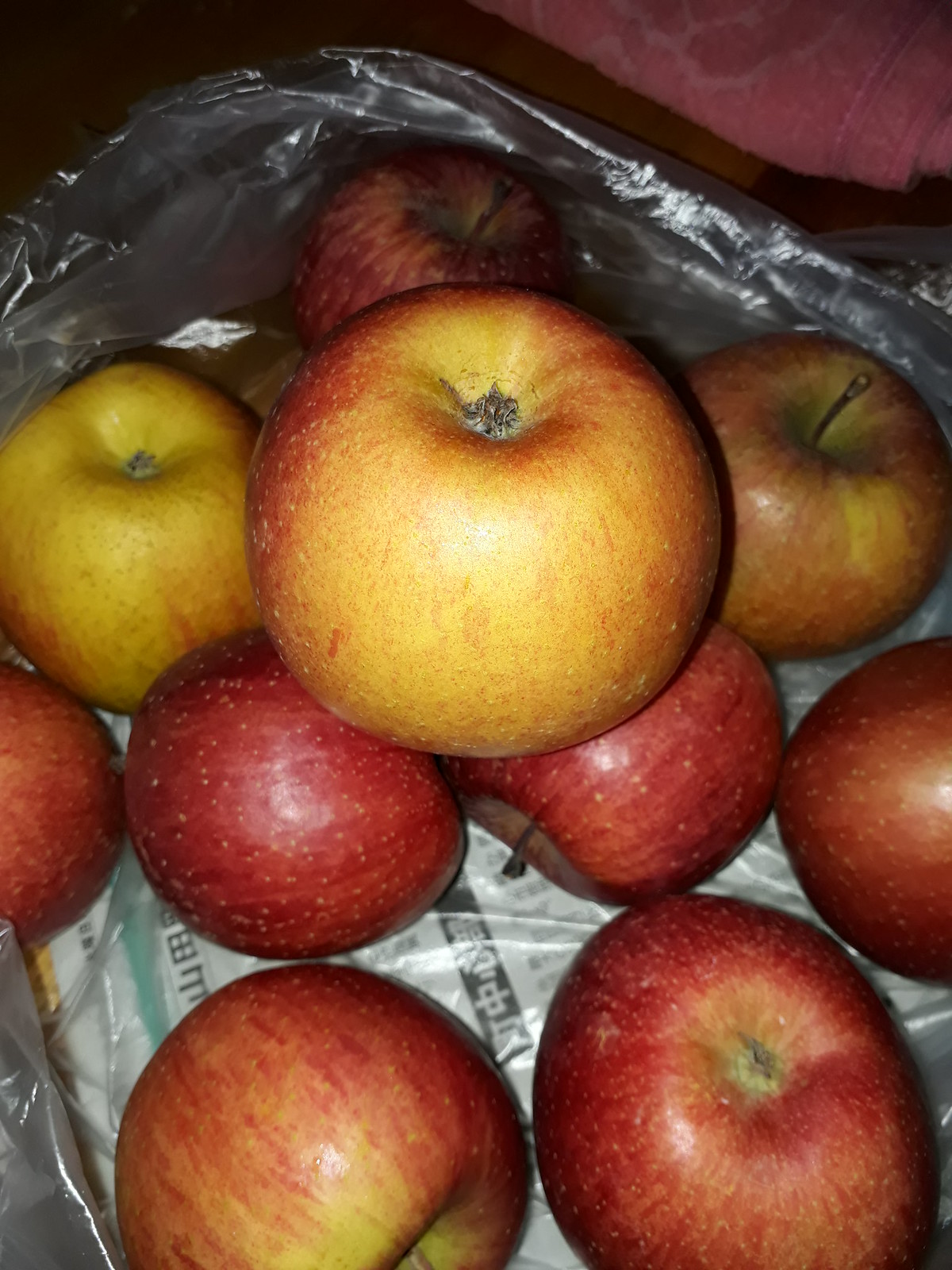This detailed photo captures a batch of apples, possibly Honeycrisp or Gala, free of any stickers, arranged haphazardly in what seems to be a clear plastic bag. The apples, exhibiting a rich red hue with some gold accents, are significantly large, approximately the size of a woman's hand. They are resting atop a layer of aluminum foil or an aluminum baking dish, which is further lined with a plastic sheet. Underneath the plastic, there appears to be a piece of paper with printed text that resembles Chinese script, hinting at the image's possible origin. The arrangement of the apples is casual, with some oriented sideways, upside down, and one positioned perched atop the others. Above the apples, a folded pink towel or dark rose-colored tablecloth is visible, extending out of the upper right corner of the image. The background is a dark wooden table, though it is obscured, giving prominence to the apples under the camera’s spotlight.